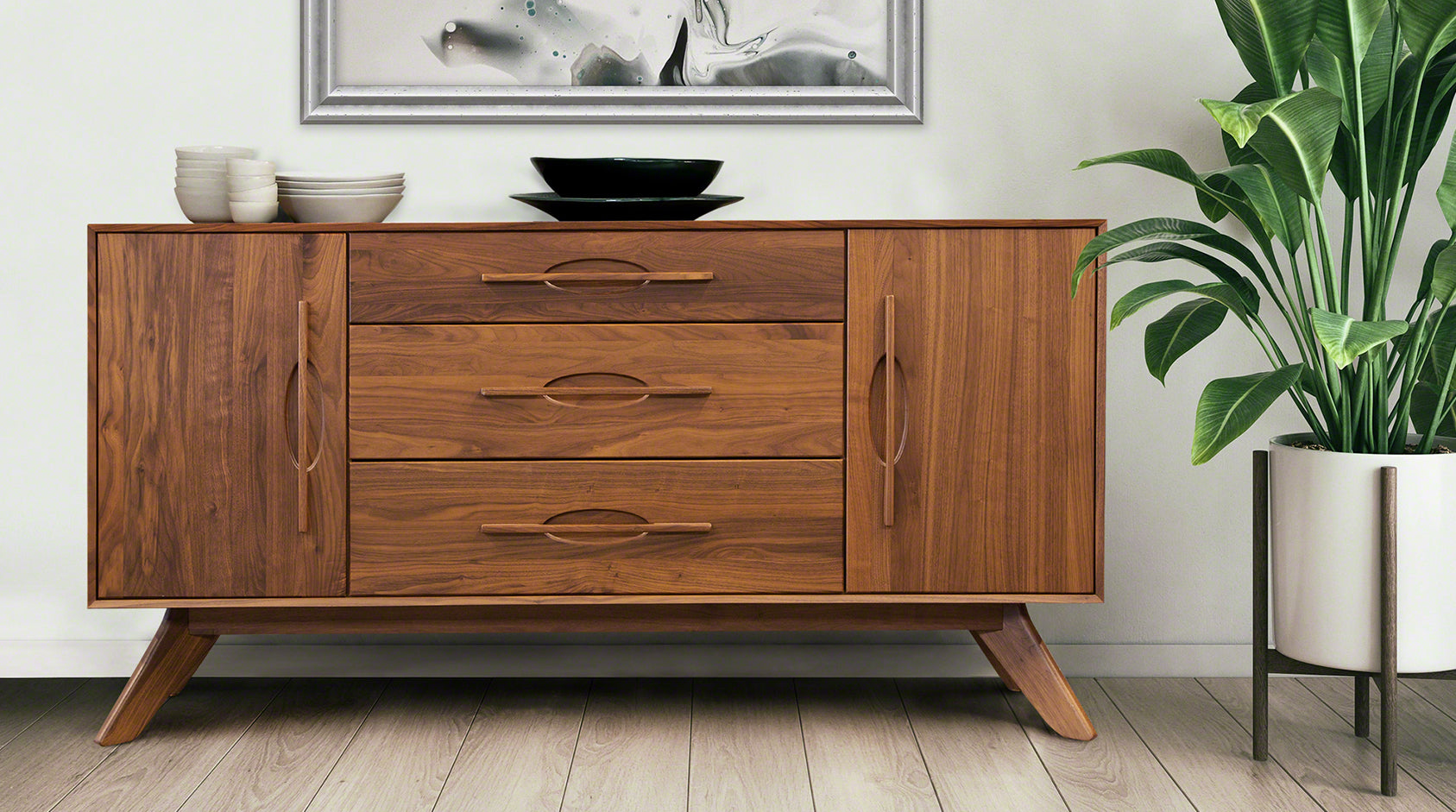In the image, we see a stylishly decorated room with a vintage 1940s-1950s wooden buffet positioned against a white wall. The buffet, characterized by its medium-brown wood tone and angled legs, features two cabinet doors on the left and right sides and three central drawers, all equipped with wooden handles. It sits atop a floor composed of vertically patterned, light gray wood tiles. On the buffet's surface, a collection of ceramic dishes is neatly arranged, including stacks of both white and black plates and bowls. To the right of the buffet stands a tall, vibrant green floor plant, housed in a white ceramic pot supported by a light brown wooden stand. Above the buffet, a partially visible silver picture frame contains an abstract, marbled black and white artwork, adding an artistic touch to the scene. The overall aesthetic is clean and harmonious, with a blend of vintage charm and modern decor.